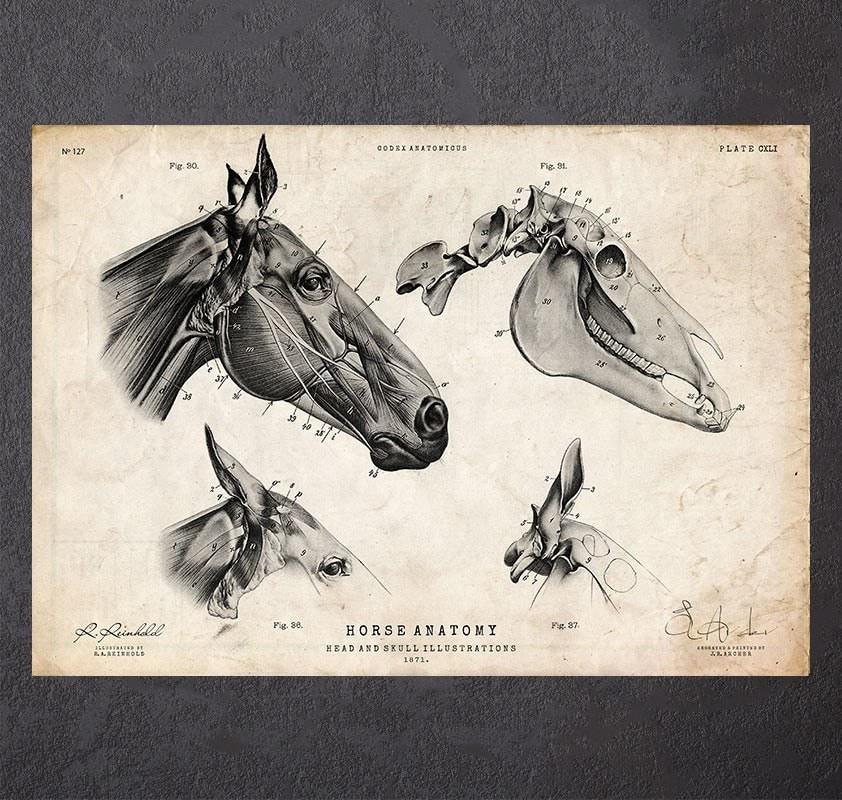This black and white vintage poster from 1871 provides a detailed examination of horse anatomy, focusing specifically on the head and skull. The poster features several intricate illustrations: the main image depicts the horse's muscles, including the ears and eyes, with various parts meticulously labeled. The skull of the horse is shown to the right with a similarly detailed breakdown, featuring numbered labels connected by arrows pointing to specific bones. At the bottom, there are additional close-up illustrations of the horse’s head, ear muscles, and bone structure, marked as figures 30, 36, 37, 90, and 91. Latin text appears at the top. The poster includes two signatures—one in the bottom right and another in the bottom left. The title reads: "Horse anatomy, head and skull illustrations, 1871," suggestive of its scientific purpose. The paper appears aged and rundown, adding to its vintage authenticity.